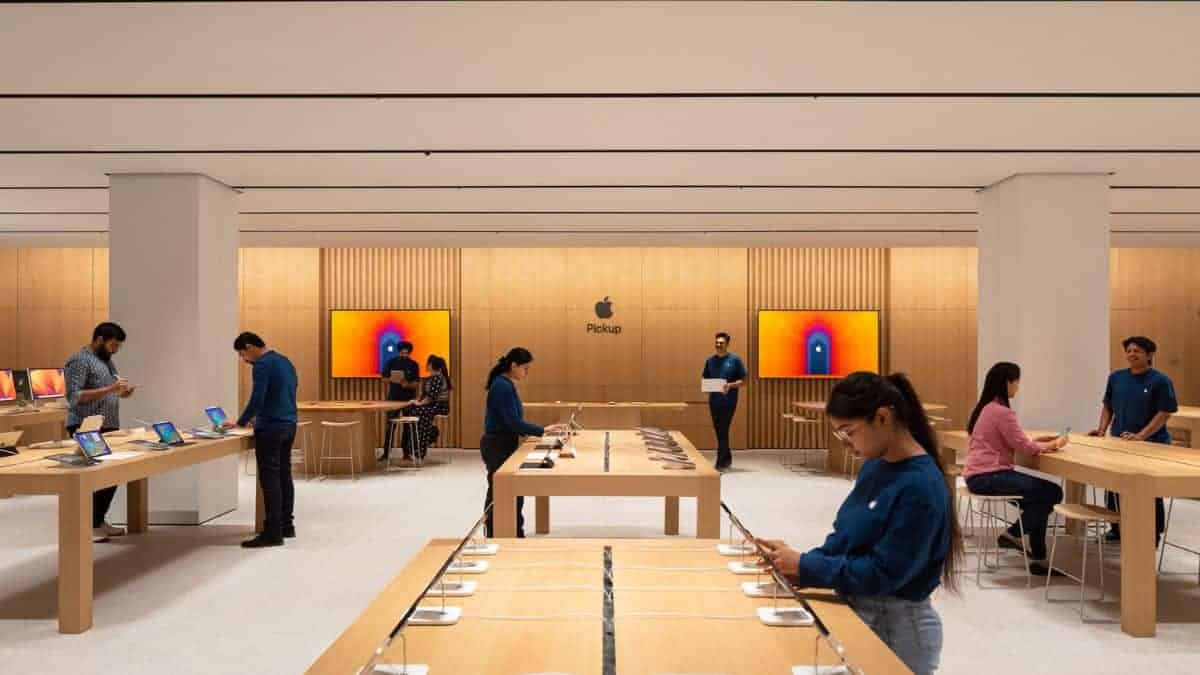In this detailed indoor scene, an Apple Store's pickup area is depicted with a focus on rows of long tables, each equipped with around a dozen tablets. The room is characterized by its modern design elements, including two imposing pillars and a white ceiling accentuated by black lines, which appears low from the given angle. The background features a wooden wall prominently displaying the "Apple Pickup" sign. Two large digital screens behind the tables show vibrant yellow backgrounds with abstract blue door designs.

The tables, surrounded by stools, host several individuals engrossed in the tablets, suggesting an interactive or product demonstration environment. Notably, a girl with a long ponytail, glasses, a blue shirt, and jeans stands at the forefront, drawing attention among the visitors. Another girl, also in a blue shirt paired with black jeans, is visible, contributing to the scene’s lively atmosphere. The presence of multiple individuals in the same blue attire, likely Apple employees, further enhances the organized and customer-focused ambiance of this Apple Store pickup area.